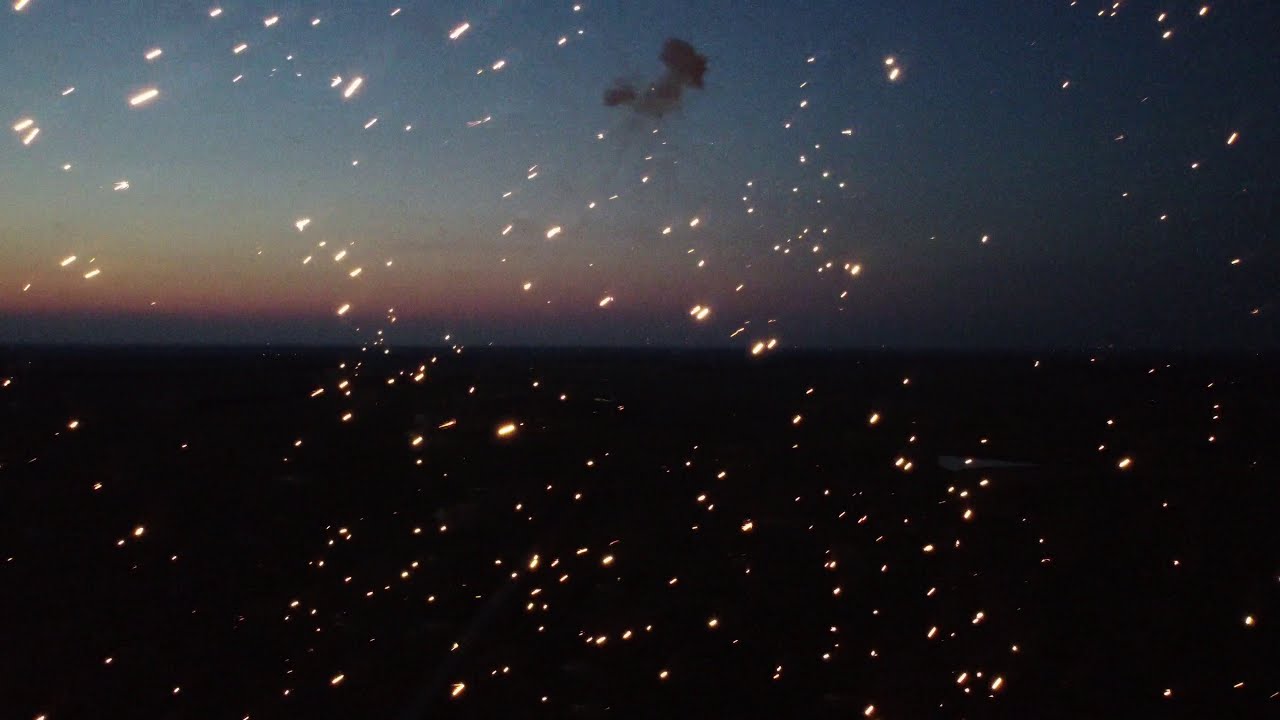This rectangular photograph, reminiscent of older, lower-quality images from around 20 years ago, displays a striking sunset horizon. In the upper section of the image, the sky transitions smoothly through bands of blue, light yellow, orange, pink, and red as the sun disappears below the horizon, casting a warm, multi-hued glow across the landscape. At the very top, a smoky cloud centers the frame, adding an ethereal quality to the scene. The bottom half of the photograph is mostly dark, suggesting that we're looking over a body of water with an indiscernible shoreline, shrouded in the night.

Scattered across the entire image are numerous tiny light specks, which closely resemble embers or sparks, creating a captivating visual effect. These sparks appear vivid and close to the camera, much like they would if one were capturing the glow from a campfire or fireworks, reinforcing a sense of warmth and intimacy. This intriguing interplay of colors, patterns, and the overlay of sparks makes the photograph both complex and fascinating, evoking a countryside night view with an almost mystical ambiance.